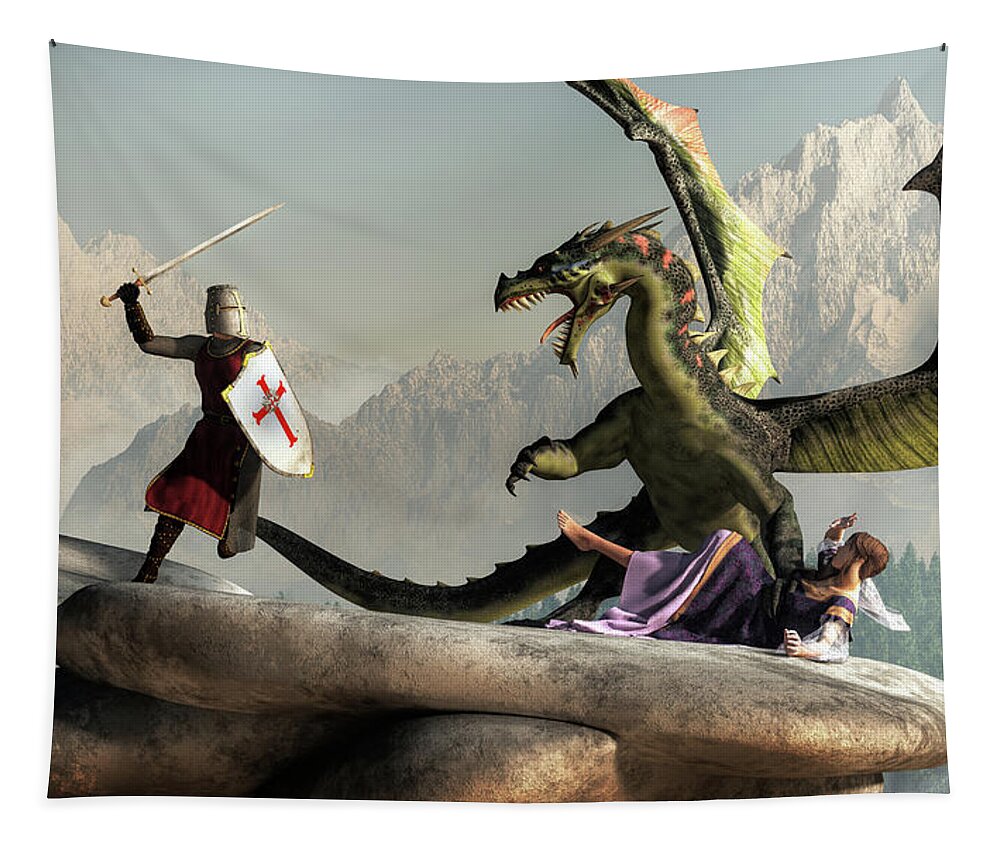This illustration, possibly created on a piece of fabric wall hanging, vividly depicts a dramatic fantasy scene. At the center is a valiant knight, garbed in silver armor with a distinctive bucket helmet. Over his armor, he wears a red tunic covering the front of his chest and legs, and he proudly holds a white shield emblazoned with a red cross. The knight, positioned on a large rock slab, faces right with his sword raised high, ready to confront a menacing green dragon. The dragon stands on its hind legs, its mouth agape revealing sharp teeth, and features dark green scales with orange stripes running along its back. Its impressive wings are spread, extending toward the top right corner of the illustration. Beneath the dragon, a barefoot woman lies sprawled on the rocky ground, dressed in a purple gown with light purple trimming. She appears distressed, covering her face with her hands. In the distance, a gray sky looms over a mountain range with snow-capped peaks, adding to the epic ambiance of the scene.